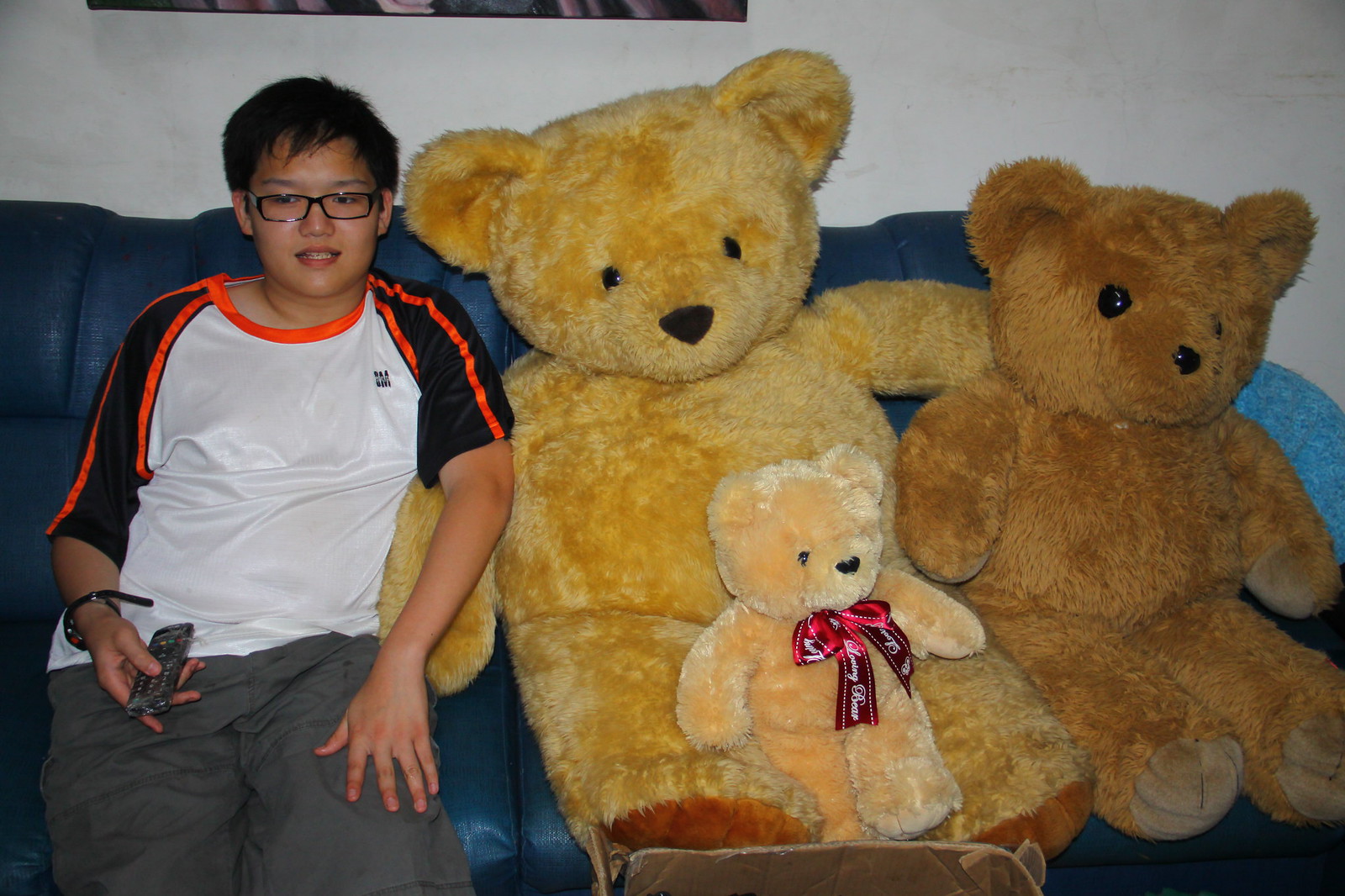In the photograph, a young Asian boy, approximately 9 to 12 years old, is seated on the left side of a blue couch positioned against a white wall. He has short dark hair and wears rectangular black glasses. The boy dons a white short-sleeved shirt with distinct black sleeves adorned with bright orange stripes and an orange neckline. In his right hand, he holds a remote control, and his right wrist sports a black watch. 

To his left side, lining up towards the center and right end of the couch, are three teddy bears of varying sizes and colors. Closest to him is an enormous, golden-colored teddy bear, almost as big as he is. Sitting on the lap of this giant bear is a smaller teddy bear with a light tan hue, distinguished by a red ribbon with white cursive writing around its neck. The third bear, positioned to the far right, is slightly smaller than the giant bear and showcases a darker brown color. All the teddy bears feature classic black eyes and a small black nose, contributing to their adorable appearance.